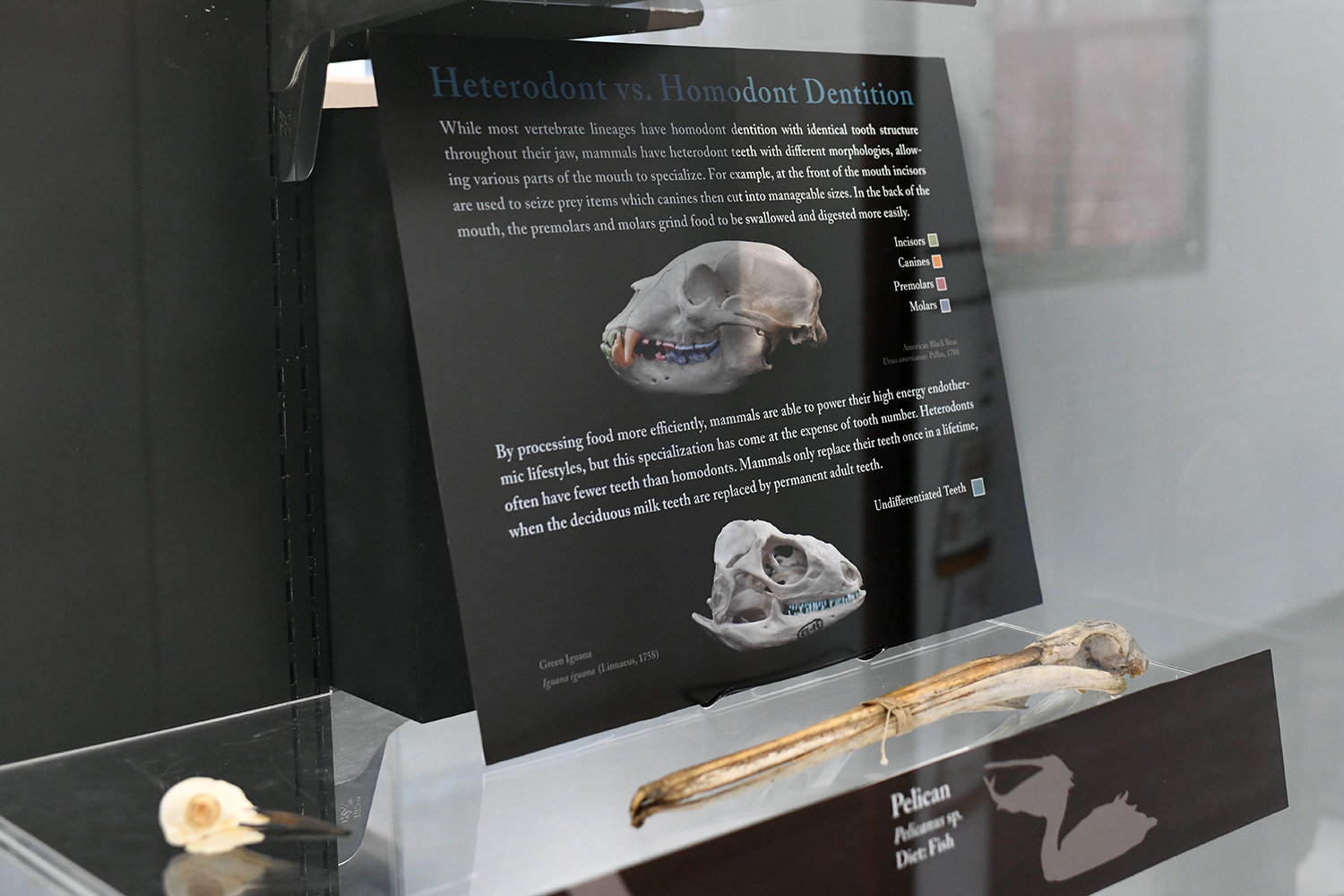The image depicts a detailed museum display focusing on the concept of heterodont versus homodont dentition. The display features a black panel, likely made of metal or plastic, with white text that explains the differences in dentition types. It highlights that while most vertebrates have homodont dentition, where teeth are uniform throughout the jaw, mammals exhibit heterodont dentition with varied tooth morphologies. This specialization allows different parts of the mouth to handle specific tasks, such as incisors at the front for seizing prey, canines for cutting, and premolars and molars in the back for grinding food. The display includes informative diagrams showing skulls and color-coded teeth: incisors, canines, premolars, and molars. It also features a skeleton and photographs of a pelican, emphasizing its unique beak structure. Additionally, there's a leg bone positioned in front of the setup, further contributing to the educational exhibit on vertebrate dentition.